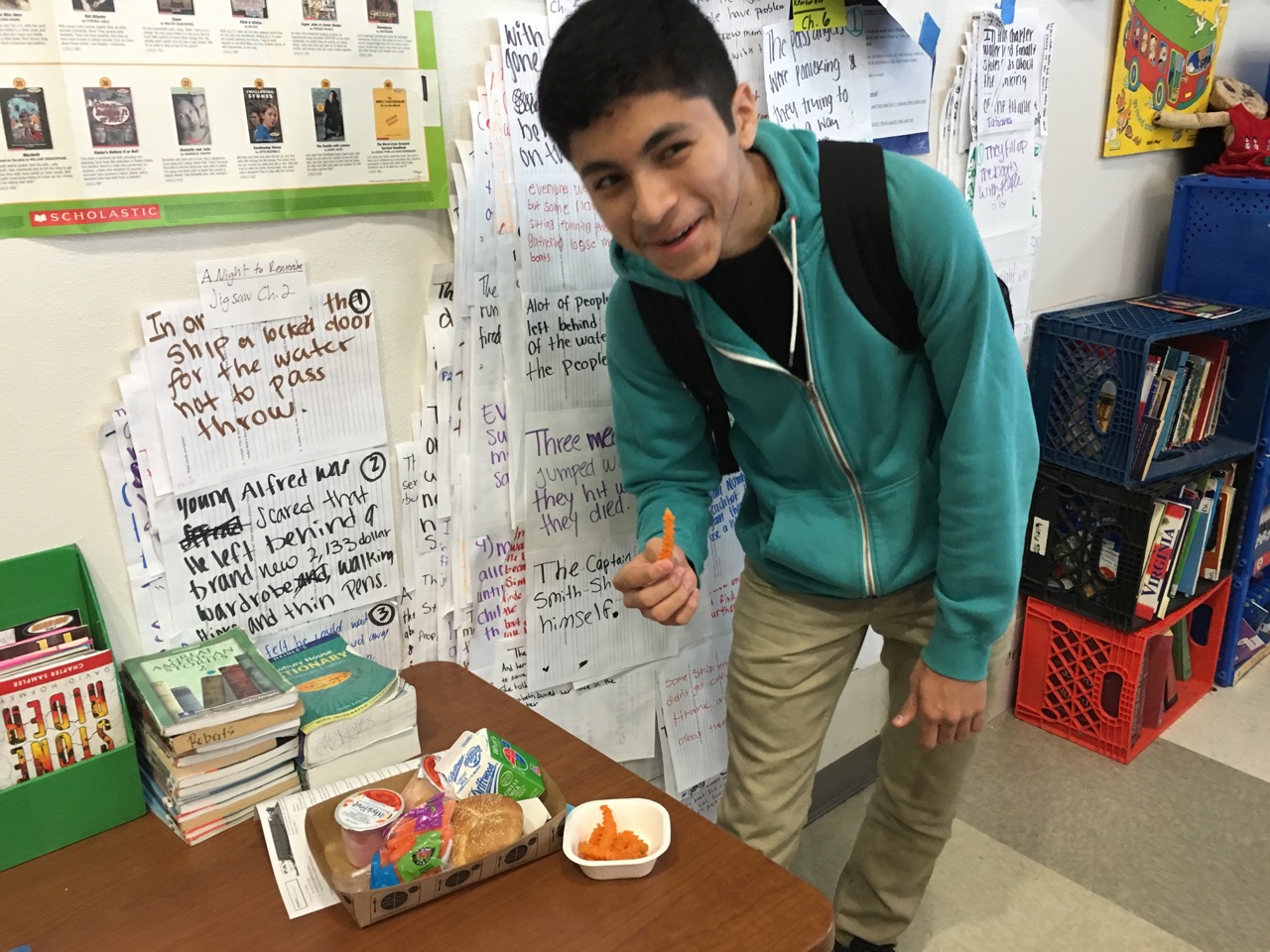In a bright and busy classroom with white walls, a young boy—estimated to be around 12 to 15 years old with short brown hair—stands beside a desk, slightly bent over as he eats a french fry from his lunch. Behind him, a blue crate, black crate, and red crate, all brimming with books, are stacked. The classroom wall is adorned with various signs, posters, and a chart displaying different books, creating a scholastic atmosphere. 

The student, wearing a green hooded sweatshirt with a white zipper and tan pants, carries a black backpack over both shoulders. On the table beside him are some books and an open green folder with more books on it. His lunch, consisting of a hamburger, milk, juice, and possibly an ice, is placed in a small box next to white container filled with fries. There is also a wrestling figure placed on one of the crates and a bus poster on the wall. The classroom's beige and tan linoleum floor reflects the organized chaos of a typical school environment. The boy appears content, smiling slightly as he savors his french fry, fully immersed in his surroundings.